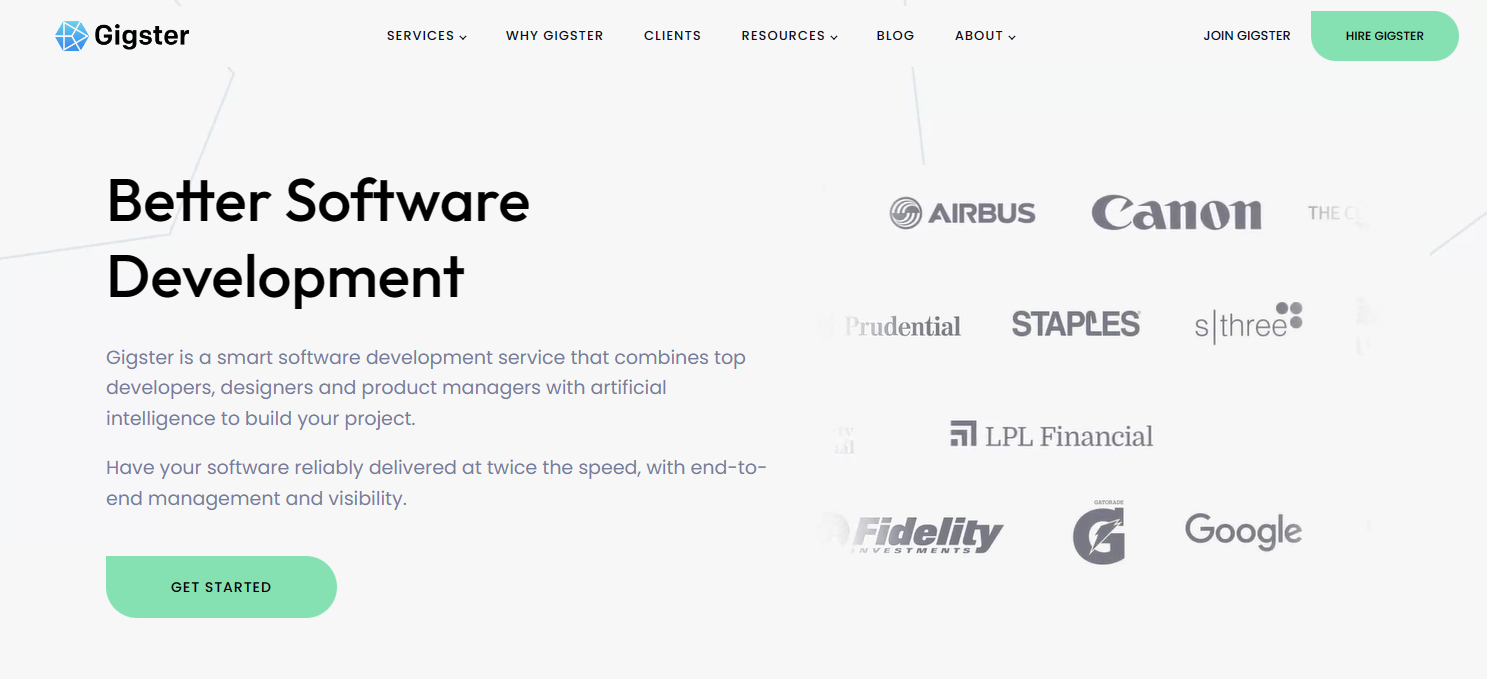**Screenshot of Gigster Website Interface**

In the top left corner, the website header features the Gigster logo accompanied by a blue circular icon. To the right of the logo, a navigation menu includes several options: 

1. **Services** (with a drop-down menu)
2. **Why Gigster**
3. **Clients**
4. **Resources** (with a drop-down menu)
5. **Blog**
6. **About** (with a drop-down menu)

In the top right corner, there's a "Join Gigster" link followed by a prominent green button labeled "Hire Gigster."

Descending from the header, the main content starts with the bold headline "Better Software Development" in black text. Below the headline, a descriptive paragraph explains that Gigster is a smart software development service integrating top-notch developers, designers, and product managers with artificial intelligence to ensure high-quality project delivery. It promises software that is reliably delivered at twice the speed, featuring end-to-end management and full transparency. A green "Get Started" button invites users to initiate their project.

On the right side of this description, corporate logos of notable clients are displayed in a list format, including:

- Airbus
- Canon
- Prudential
- Staples
- LPL Financial
- Fidelity
- Google
- Gatorade